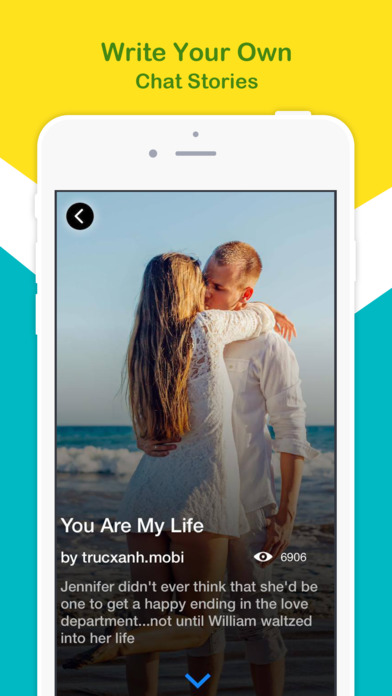The image illustrates a step-by-step guide on how to write your own chat stories. Central to the image, a romantic scene unfolds with a couple sharing a kiss on the beach under a clear sky. The tide is gently approaching the shore, adding a serene backdrop to their intimate moment. Both individuals are clad in white; the woman wears a flowing dress with her long hair cascading down her back, while the man sports rolled-up sleeves and capri pants. Hovering above them, the text "You are my life by trookexon.mobi" is prominently displayed, indicating 6,906 views.

The narrative below the main image reads: "Jennifer never thought she'd experience a happy ending in love until William waltzed into her life." All this is encapsulated within a white phone screen, with the title "Write your own chat stories" in green text against a yellow, irregularly shaped background at the top. The phone in the image is bordered with a green outline on both the left and right sides, completing the visual presentation.